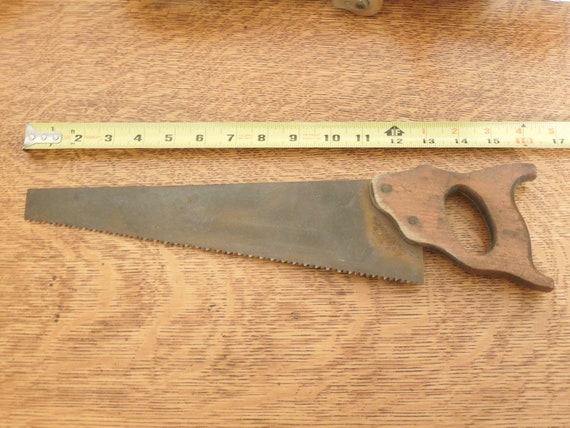This photograph captures an overhead view of an old, somewhat rusted manual handsaw placed on a wooden table with a texture that suggests a lacquered finish, characterized by blonde hues and fine dark lines. Next to the saw, a yellow metal tape measure is laid out horizontally from left to right, depicting the length of the saw for comparison. The handsaw, measured at 16 inches including the handle, has a noticeably worn wooden handle that is fixed to the blade with two metal screws. The blade itself shows signs of neglect, with blackened, oxidized areas and rust particularly evident near the handle. The overall scene suggests a setup meant for a procedural measurement or documentation, showcasing the aged state of the tool against the warm, detailed backdrop of the wooden surface.